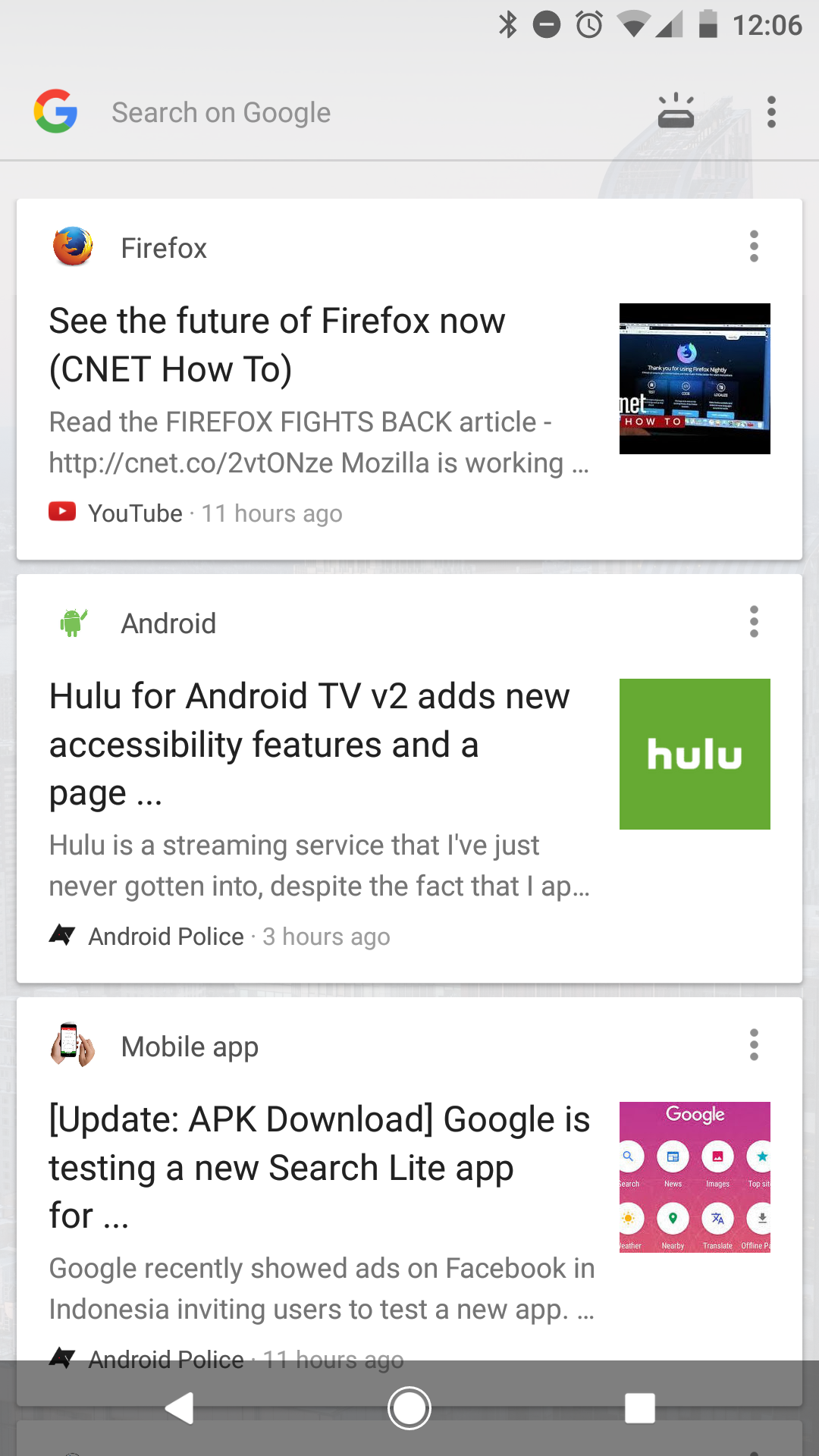**Detailed Description of the Smartphone Screenshot:**

In this screenshot from a smartphone, the interface presents three distinct app options. The background is uniformly gray. At the top right of the screen, several status icons are displayed: Bluetooth, wireless connectivity, signal strength, battery life (approximately 50%), and the current time, 12:06.

Just below these icons, the screen features the Google search bar, identifiable by the multi-colored Google "G" (red, yellow, green, and blue) and the placeholder text "Search on Google" in gray.

Immediately beneath the search bar, there are three white rectangular sections, each containing an app suggestion with a corresponding logo, title, description, and a thumbnail image on the right.

1. **Firefox:**
   - *Logo*: A planet symbol wrapped in yellow and orange hues.
   - *Title*: "Firefox" in gray font.
   - *Description*: "See the future of Firefox now (CNET). Read the Firefox Fights Back article, http cnet.co" in black text.
   - *Additional Info*: "YouTube - 11 hours ago."
   - *Thumbnail*: A mix of dark blues, light blue, red, and white lettering depicting some visual content from YouTube.

2. **Android:**
   - *Logo*: A green icon of a robot-like creature.
   - *Title*: "Android" in gray font.
   - *Description*: "Hulu for Android TV v2 adds new accessibility features and a page" in black text.
   - *Thumbnail*: A green rectangle with "Hulu" written in white.

3. **Mobile App:**
   - *Logo*: An image of a mobile phone held vertically.
   - *Title*: "Mobile App" in gray font.
   - *Description*: "Update APK download. Google is testing a new Search Lite app for..." in black text.
   - *Additional Info*: "Android Police - 11 hours ago" in gray, accompanied by a black symbol.
   - *Thumbnail*: A pink square with white lettering "Google" at the top and eight different white circles with icons in various colors (blue, red, yellow, and gray).

At the very bottom of the screenshot, there's a transparent gray band featuring the standard three smartphone navigation icons in white.

This detailed description encapsulates the entire layout, down to the specifics of each section, highlighting the app options and their respective visual elements.